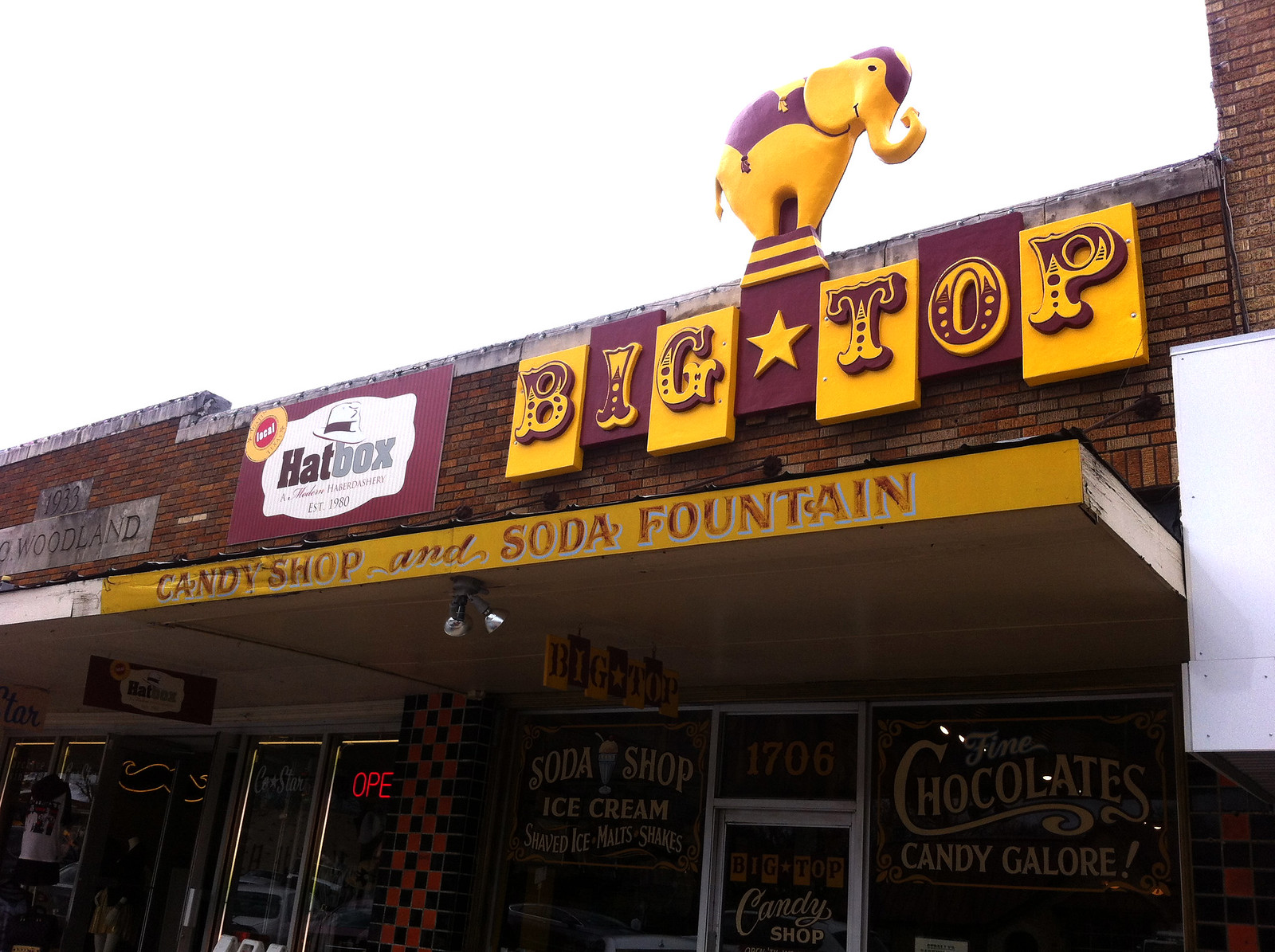The image captures the charming facade of a brick-built business park featuring multiple establishments. Dominating the scene is "Big Top," a candy shop and soda fountain, with its prominent maroon and gold signage. Above the sign, a yellow elephant with purple trim adds a whimsical touch. Below the main signage, additional text reads "Candy Shop and Soda Fountain," with storefront windows displaying phrases like "Chocolates and Candy Galore" and "Cursive Candy Shop." To the left of Big Top is another store named "Hat Box," and another establishment with partially legible writing, possibly "1993 Woodland." The setting suggests a quaint main street, and the overall visual theme is maintained with neon orange signs and a nostalgic, colorful palette.